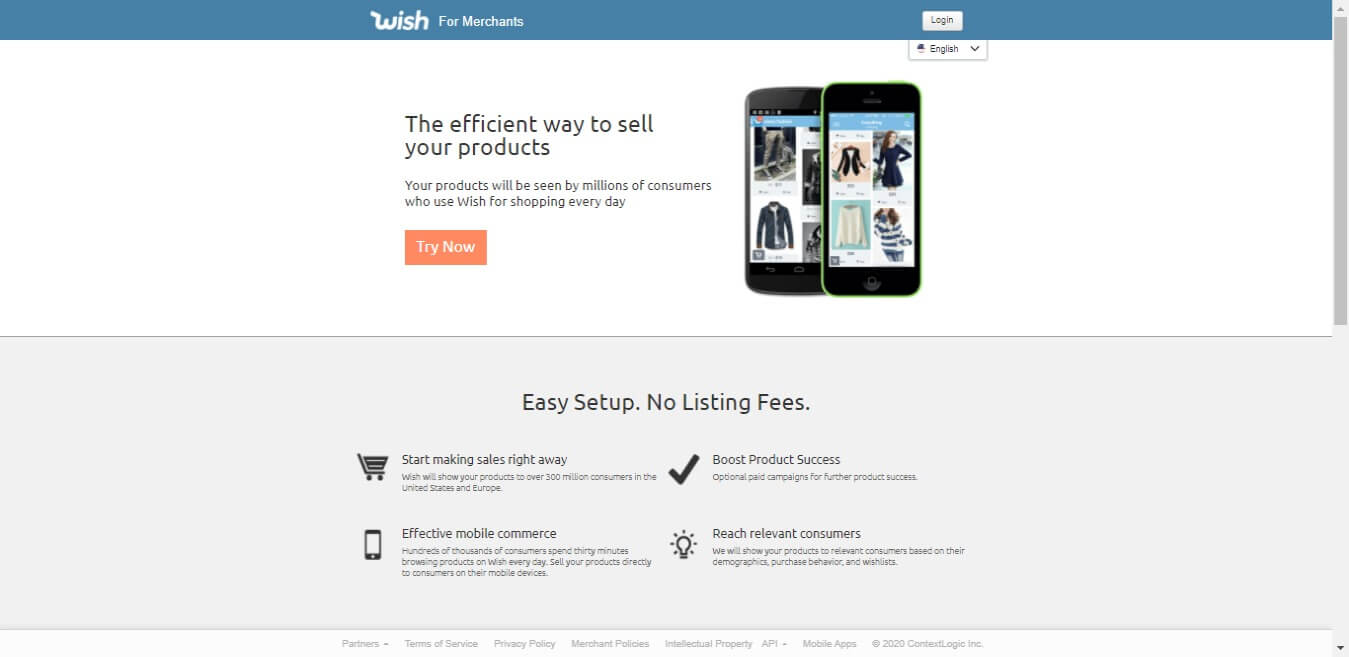Under the heading "Websites", the image displays the Wish for Merchants login page. At the top, a blue bar features the "Login" option prominently. Below it, within a white area, the language is set to English via a drop-down menu.

The central text reads, "The efficient way to sell your products. Your products will be seen by millions of consumers. Use Wish for Shopping every day. Try now." Two cell phones are showcased, each displaying images of various clothing items available for purchase online.

Further down, key selling points are highlighted: 
- "Easy setup, no listing fees" accompanied by a shopping cart icon with the message "Start making sales right away."
- "Wish will show your products to over 100 million consumers in the United States and Europe."
- "Effective mobile commerce" represented by a cell phone icon.
- "Boost product success" next to a check mark symbol.
- "Reach relevant consumers" paired with a light bulb icon. 

Additional text is present, though too small to read. The "Try now" button is orange with white text, while the "Login" button is white with black text. All other text on the page is in black print.